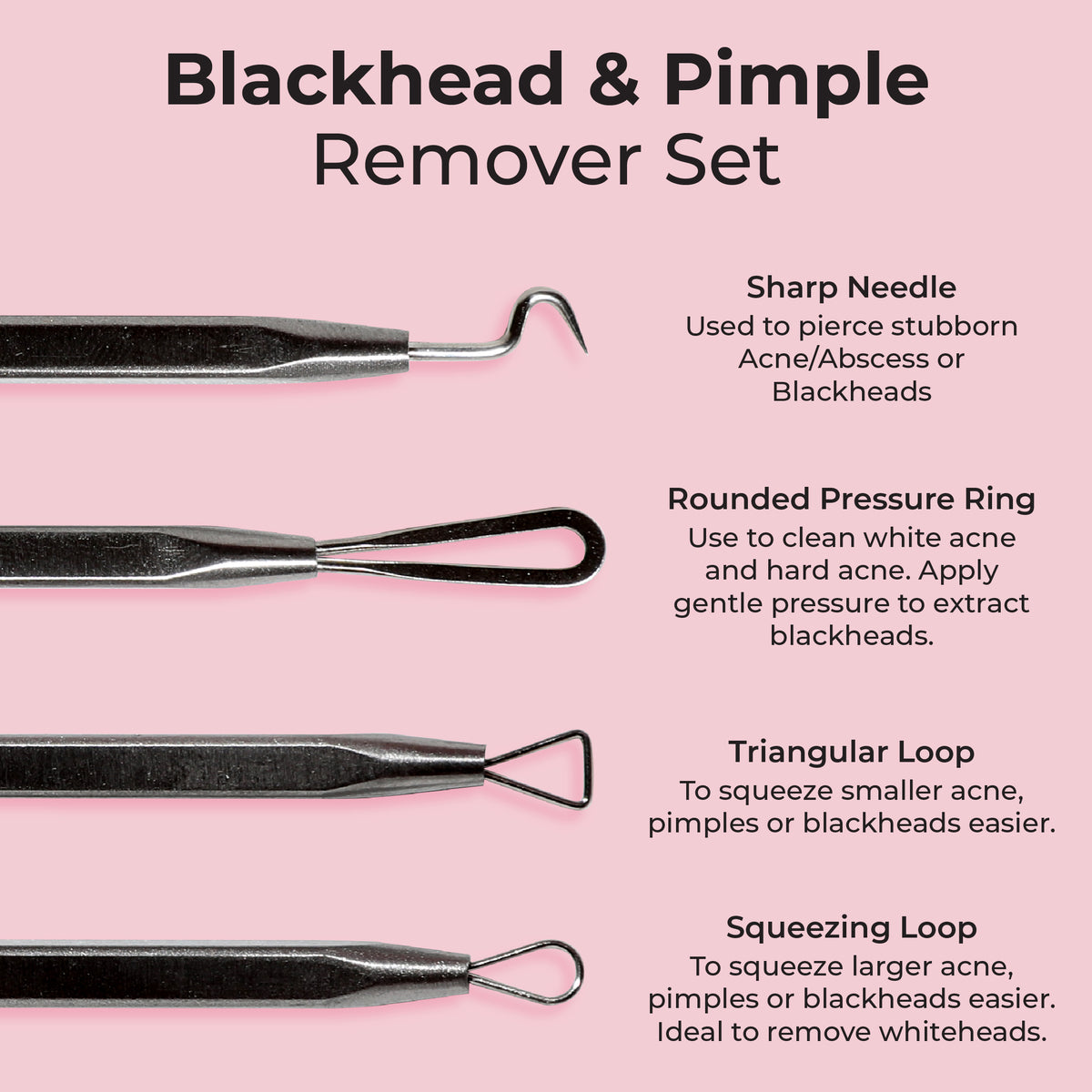The image features a pink display with a solid pink background and black text. At the top, bold font reads "Blackhead and Pimple Remover Set." To the right, various tools and their descriptions are listed: "Sharp Needle," "Rounded Pressure Ring," "Triangular Loop," and "Squeezing Loop." To the left, there are illustrations of the metal tools with detailed uses:

- **Sharp Needle:** Used to pierce stubborn acne, abscesses, or blackheads.
- **Rounded Pressure Ring:** Used to clean white acne and hard acne; apply gentle pressure to extract blackheads.
- **Triangular Loop:** Ideal for squeezing smaller acne, pimples, or blackheads with ease.
- **Squeezing Loop:** Designed for squeezing larger acne, pimples, or blackheads; perfect for removing whiteheads.

Each tool is clearly labeled and described, making it easy to understand their specific functions.